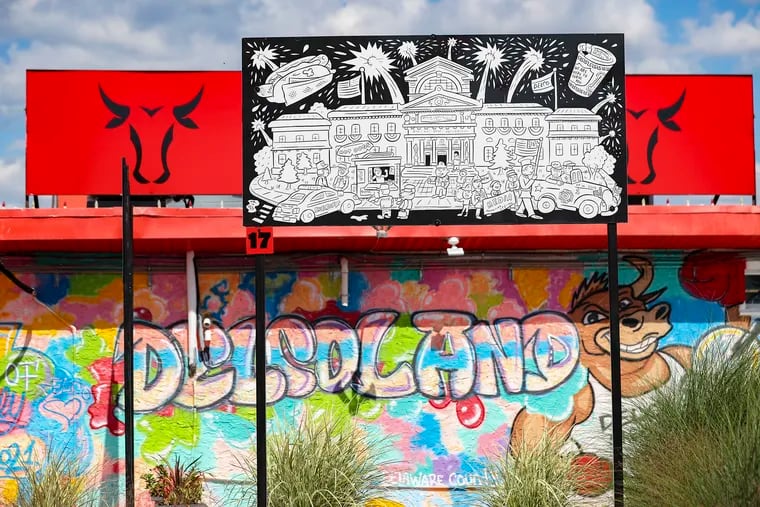The photograph captures a vibrant graffiti scene on the side of a building. Central to the image is a colorful graffiti piece that reads "Delco Land" in bold, multi-colored text featuring hues of pink, blue, green, red, and lime green. Prominently displayed in the graffiti is a character resembling a bull, which is brown with two horns, large nostrils, and a broad, toothy grin. The bull is depicted wearing a white tank top and red boxing gloves, exuding a powerful presence on the wall. Surrounding the "Delco Land" graffiti, partially obscured by five green bushes, is additional text that appears to be "Beware Council," though it's somewhat unreadable due to the foliage.

Above this graffiti, the photograph includes more artwork: a red sign with a bull symbol and the number 17, adjacent to a black-and-white painting or drawing of a city scene featuring cars, people, and fireworks. The upper background of the scene is a cloudy blue sky, adding depth to the setting. Overall, the image is a lively blend of urban street art, characterized by a mix of vivid colors and intricate details, set against the natural elements of the surrounding vegetation.